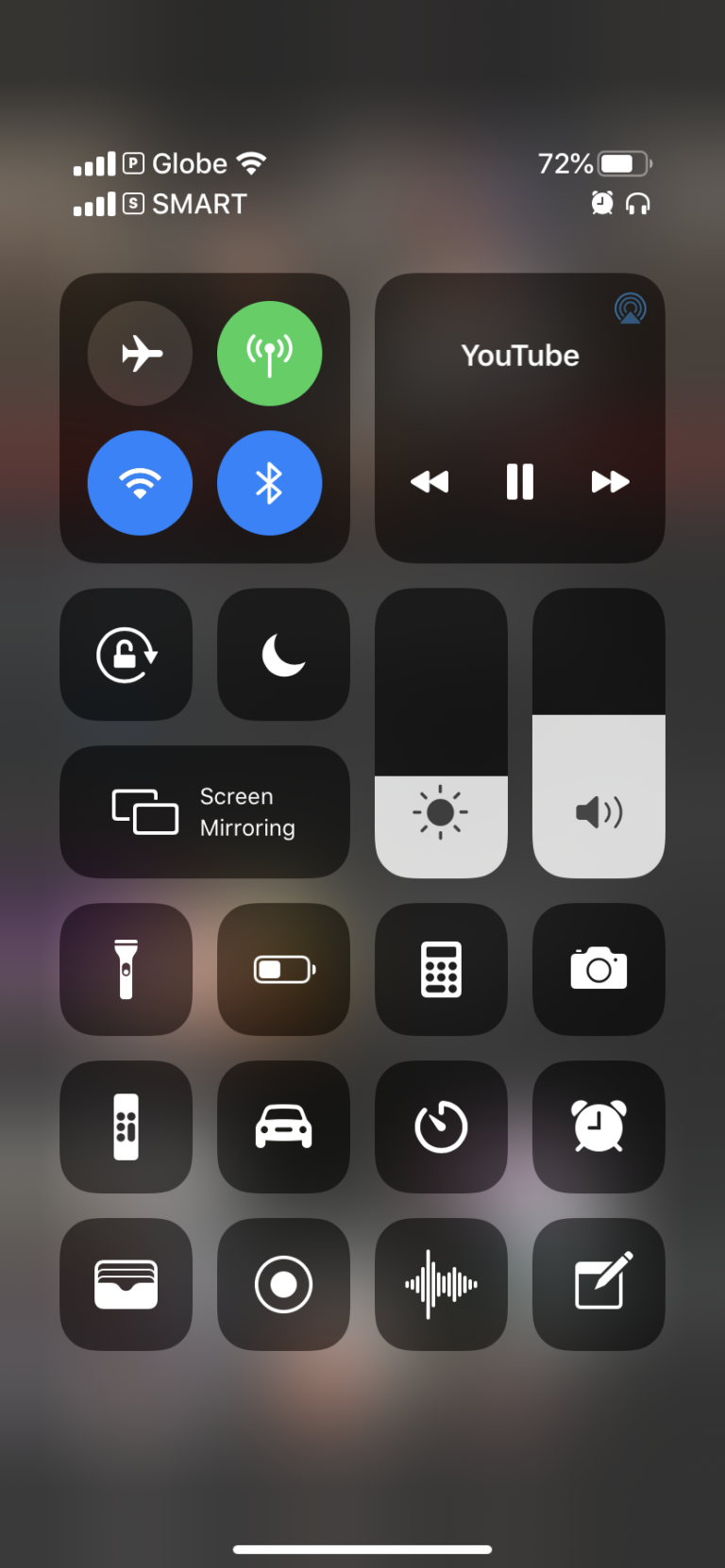A detailed screenshot of a phone menu with a partially transparent gray background. The transparency varies, with a darker shade at the top and a more translucent middle, revealing a subtle white hue beneath. On the left shows connectivity icons, displaying signal bars for "P-Globe" and a Wi-Fi symbol. Additional icons below include more signal bars, an "S" in a square, and "SMART." The battery is 72% charged, and a timer is set. To the right of the clock icon is a headphone symbol, indicating headphones are plugged in. 

The menu is symmetrically organized, with two rectangles at the top. The right rectangle features YouTube controls, including forward, pause, and back buttons. The left rectangle contains Wi-Fi and airplane mode toggles. Various buttons are arranged vertically, such as the flashlight, a yellow sound control button, and a brightness control. The layout is clean, simple, and visually balanced, with a line across the bottom for navigating to another page on the phone.